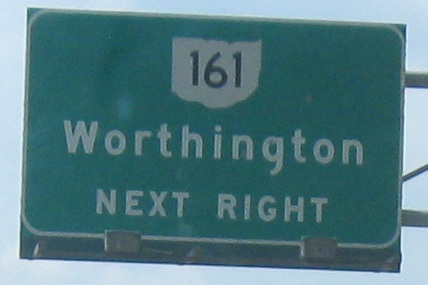This close-up photo captures a large green road sign typically found over highways. The sign dominates most of the image and is specifically for the place Worthington, with the words "Next Right" written underneath in white lettering. Above "Worthington" is a highway symbol featuring the number 161 in black on a distinctive white shape that could represent a state outline. The bottom edge of the sign is equipped with two grey floodlights which illuminate it at night. The sign is supported by a metal structure, visible to the right-hand side of the image, which includes bars and a cage-like rigging. The sky in the background is pale blue and cloudless, providing a clear backdrop for the green sign.